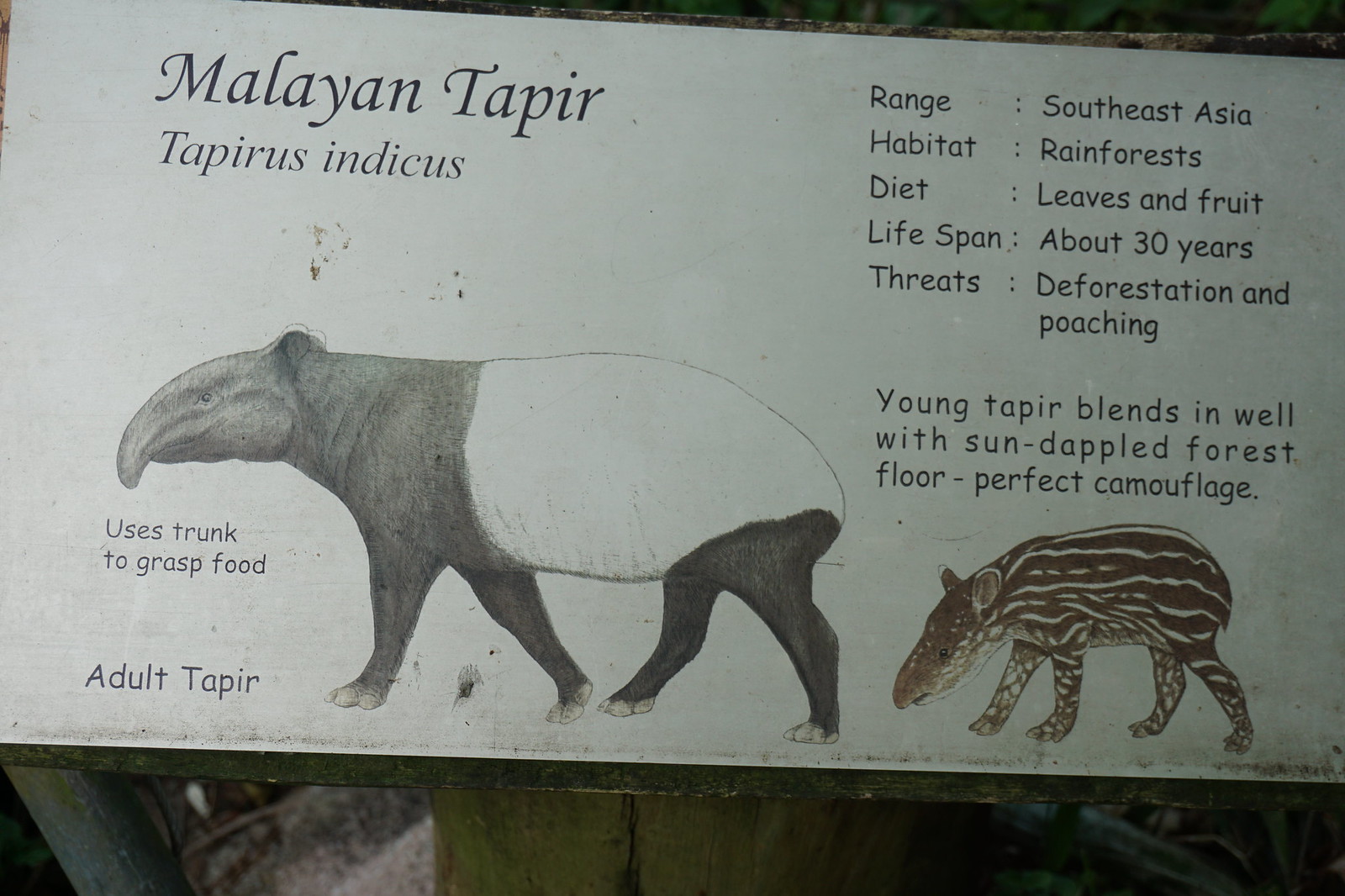The image shows an informational zoo sign about the Malayan tapir (Tapirus indicus). The sign features bold lettering and includes photographs of both an adult and a young tapir. The adult Malayan tapir is depicted in black and white, resembling a sheep in size and somewhat like a panda due to its coloration. The juvenile tapir, which is brown with white stripes and spots, exhibits perfect camouflage for the sun-dappled forest floor. The text surrounding these images provides details such as the tapir's habitat in Southeast Asian rainforests, their diet consisting of leaves and fruit, and their approximate lifespan of 30 years. It also mentions the tapir's use of its trunk to grasp food. Additionally, the sign highlights threats to the species, including deforestation and poaching, and notes that the young tapir's coloration helps it blend well into its surroundings. An outdoor post and rough wood frame the sign, indicating its placement in a naturalistic zoo setting.